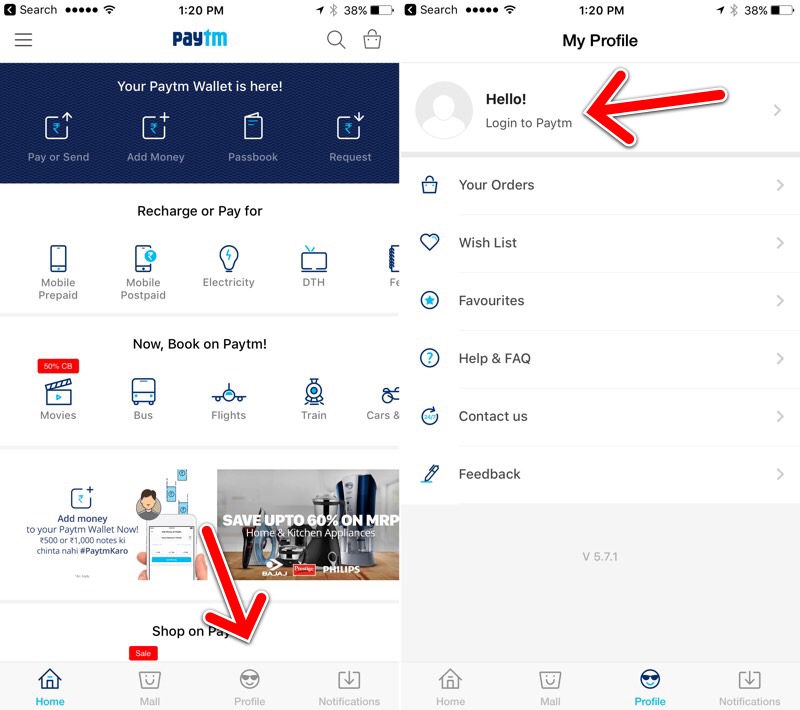The image features two side-by-side screenshots from a mobile phone, each depicting different sections of the PayTM app. At the top of the first screenshot, the PayTM logo is prominently displayed with a message indicating, "Your PayTM wallet is here." Below this, a blue bar offers several options including 'Pay or Send,' 'Add Money,' 'Passbook,' and 'Request.' Beneath the blue bar, on a white background with black text, are quick access links for various services: 'Recharge or Pay for Mobile Prepaid,' 'Mobile Postpaid,' 'Electricity,' and 'DTH.' An icon on the right side is partially visible but cut off. Further down, a section says, "Now book on PayTM," followed by truncated options like 'Movies,' 'Bus,' 'Flights,' 'Train,' and 'Cars.'

In the bottom left corner of the screenshot, there is a button labeled 'Add Money.' An advertisement is present below this button, promoting a sale with the message: "Save up to 60% on MRP home and kitchen appliances." Along the bottom of the first screenshot are navigation options, including 'Home,' 'Mall,' 'Profile,' and 'Notifications.' A red arrow superimposed on the image points to 'Profile' at the bottom of the screen.

The second screenshot displays the 'My Profile' section of the PayTM app. It greets the user with "Hello," and a prompt to "Log in to PayTM," highlighted by another red arrow pointing to the login area. Below the prompt, a list of options is presented: 'Your Orders,' 'Wish List,' 'Favorites,' 'Help and FAQ,' 'Contact Us,' and 'Feedback.' This screen also shows the app version number, '5.7.1.' Similar to the first screenshot, the bottom navigation bar includes icons for 'Home,' 'Mall,' 'Profile,' and 'Notifications.'

This detailed descriptive caption provides a comprehensive overview of the elements within each screenshot, emphasizing navigation options, promotions, and user prompts within the PayTM application.